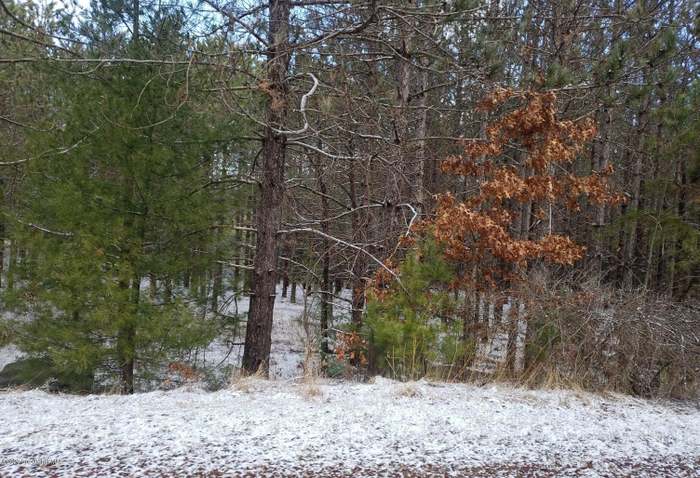A serene winter scene unfolds in this horizontal photograph of a forest. The foreground is a snowy stretch of land with patches of brown dirt peeking through, suggesting a recent, light snowfall. Dominating the midsection are a variety of trees, predominantly leafless and displaying their wiry, gray and brown branches. Among them stands a prominent bare tree with long, twisty branches, adding a dramatic element to the landscape. To its right, a smaller, yet vibrant green fir tree contrasts against the otherwise stark scenery.

Adjacent to this fir tree is a deciduous tree, smaller in stature, still clinging to its brown leaves, providing a faint hint of life amid the wintry barrenness. Throughout the forest, there are scattered evergreens, particularly concentrated on the left side of the image, and growing closely together, contributing a splash of green. These evergreens intermingle with the branches of bare trees, creating an intricate tapestry.

In the background, bits of the muted blue sky are visible through the gaps in the canopy, hinting at a cloudy but not entirely overcast day. A small berm covered in snow can be seen towards the front, edged by sparse brown bushes on the right, their leafless stems forming a low-lying brush.

Overall, the image captures the tranquil yet desolate beauty of a forest in winter, with hints of green from the evergreen firs adding color to the monochromatic palette of gray branches and white snow.